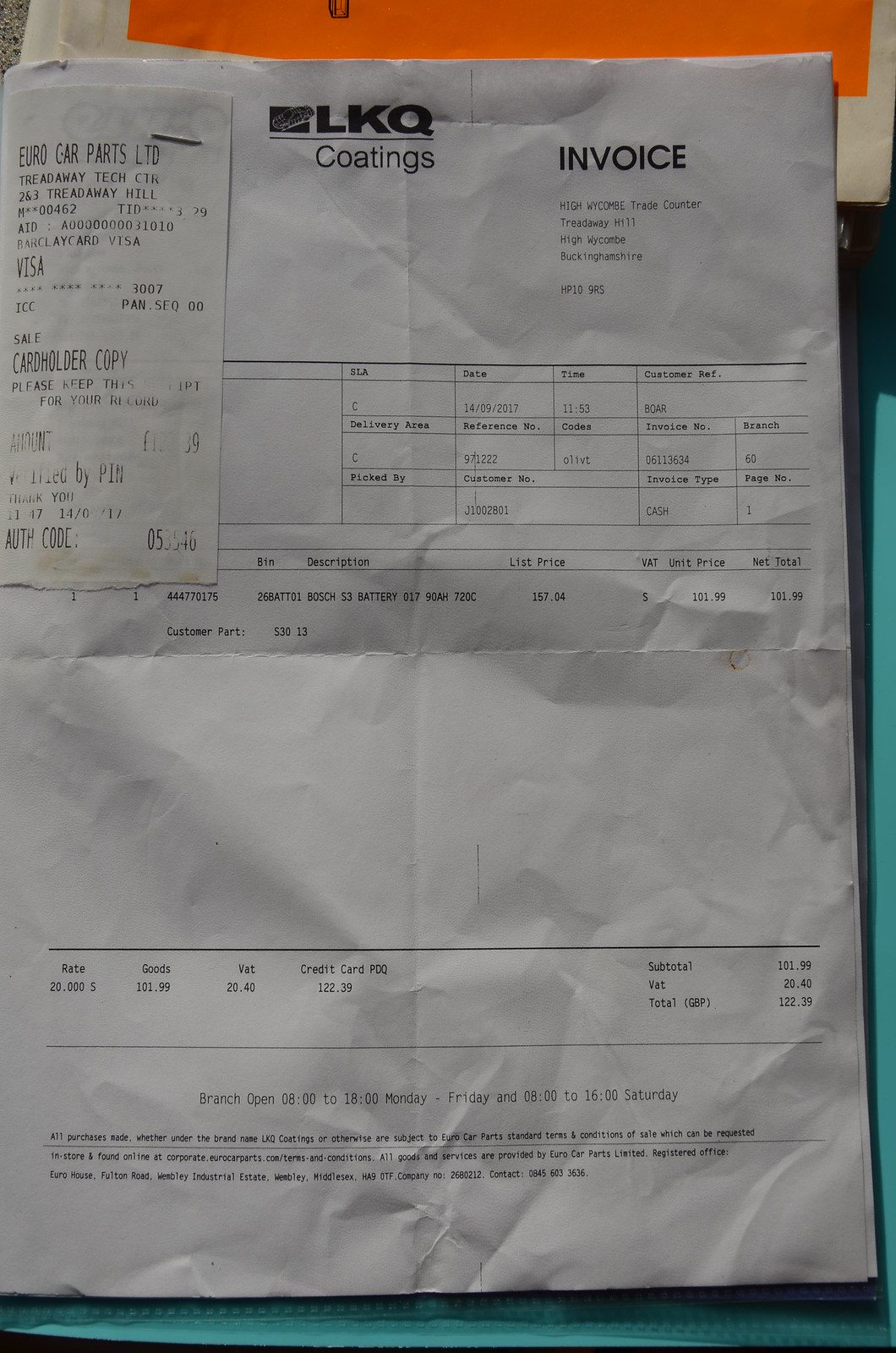The image depicts a rectangular photograph that is roughly twice as tall as it is wide. The main focus of the image is an invoice from "LKQ Coatings," occupying about 90% of the space, printed on white, quadrantly-folded paper. The top of the image features a neon orange rectangular area, beneath which the invoice is visible. "LKQ" is printed in large black bold letters, followed by a non-bold "Coatings" below a thin black divider. To the right, "INVOICE" is also prominently displayed in black capital letters. An attached receipt is stapled to the left side of the invoice, reading "EUROCARPARTSLTD TREADAWAY TECH CENTER," with "CENTER" abbreviated as "CTR". The receipt outlines various transaction details such as rates and payment amounts, including terms like "RATE 20.000S," "GOODS 141.99," "VAT 23.40," "CREDITCARD PDQ 122.99," "SUBTOTAL 101.99," "VAT 20.40," and "TOTAL GBP 122.39". The background of the photo includes a teal-colored surface at the bottom and right, along with an off-white paper material underneath the invoice and an additional square piece of teal paper at the top.